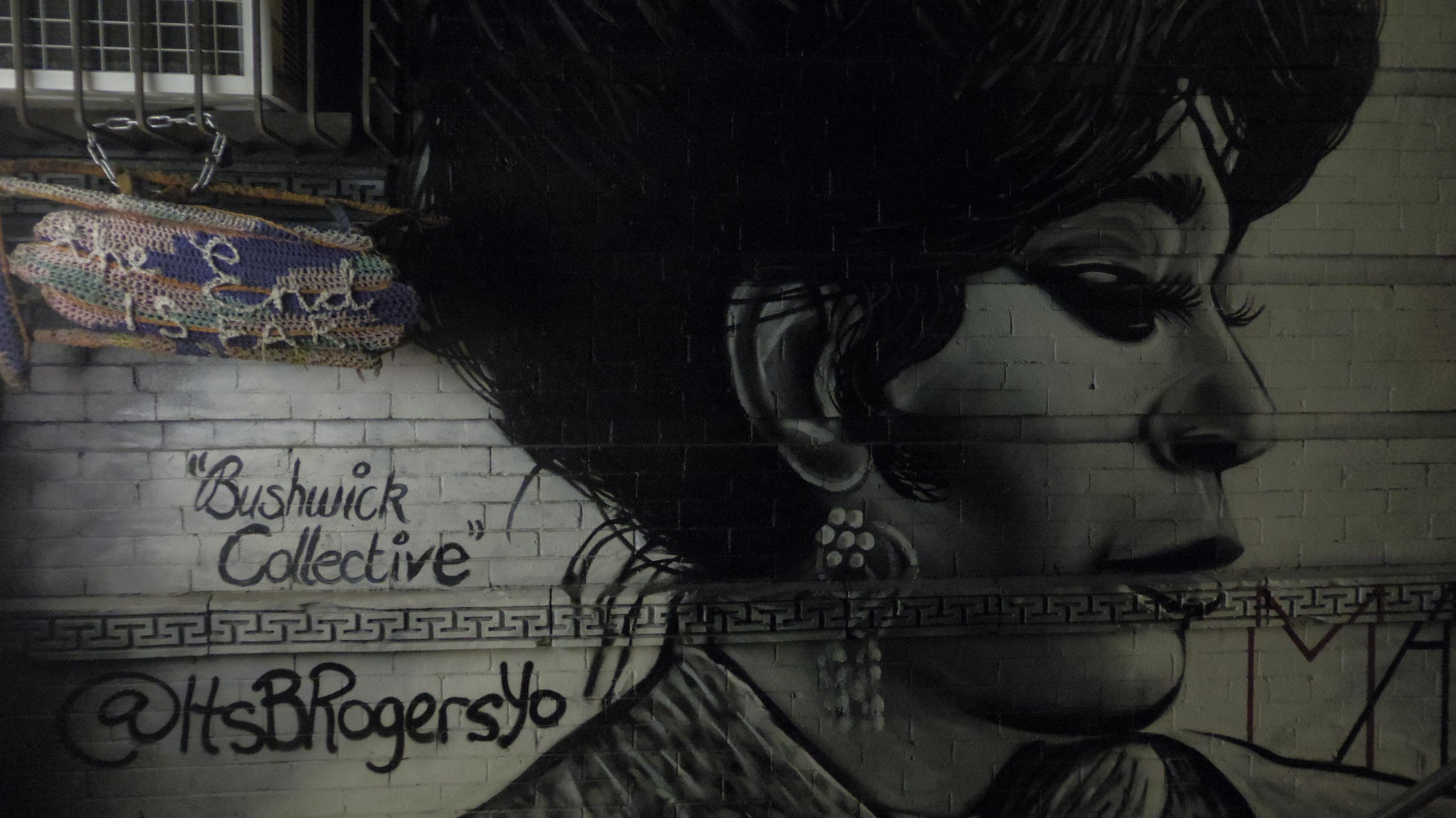The image depicts an artfully graffitied brick wall, painted a cream color. Dominating the scene is a detailed side profile of a woman with dark hair elegantly pulled up, long eyelashes, and dangly earrings, her lips suggesting a soft and friendly smile. The artwork is set against a dimly lit backdrop that blurs the line between exterior and interior. In the top left corner, part of an air conditioning unit, encased in bars and adorned with a colorful crocheted item on a chain, bears the embroidered words "the end is near." Below, black graffiti includes the text "Bushwick Collective" with "at HSB Rogers Yo" inscribed, though interpretations vary slightly. The scene also features graffiti initials "M.A." in the bottom right, adding to the monochromatic yet artistically rich portrayal.